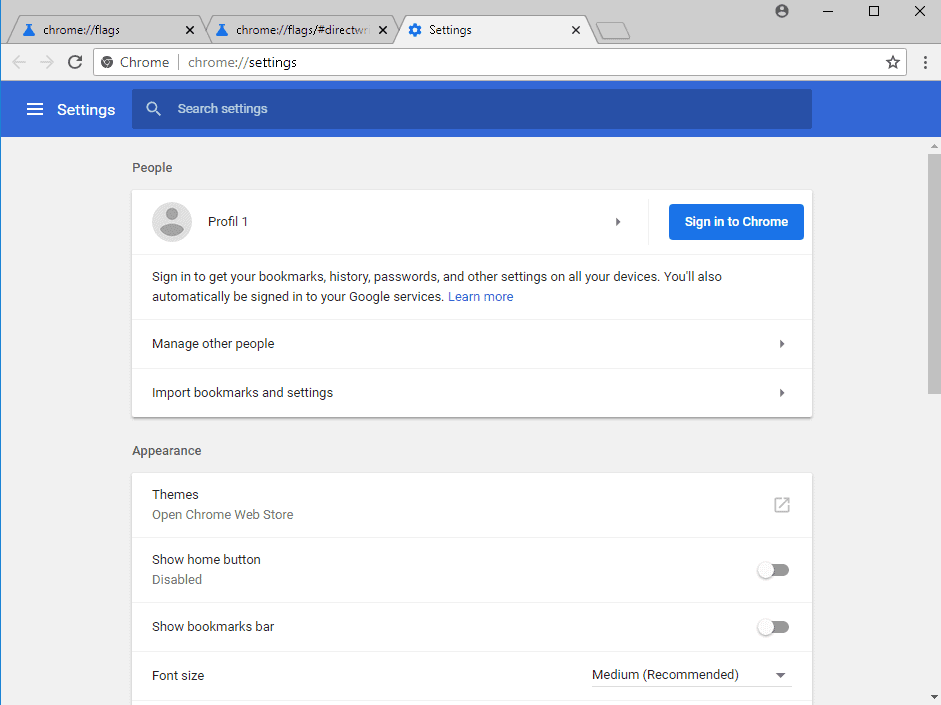A detailed screencap of a Google Chrome settings page, displayed through an open tab that is highlighted in white and reads "Settings". The address bar reflects the URL "chrome://settings." To the left of this highlighted tab are two other tabs: one labeled "chrome://flags" and another with the URL "chrome://flags/#direct."

The header banner at the top of the page is blue, with the word "Settings" in white text on the far left. Next to "Settings" is a dark blue search bar containing the text "Search settings" in white, along with a magnifying glass icon.

The main content of the settings page is divided into sections, each with a white background against a light gray page. The first section is titled "People." Within this section, the user is identified as "Profile 1," with a blue button labeled "Sign in to Chrome" next to it in white text. Below this, there is a message that reads: "Sign in to get your bookmarks, history, passwords, and other settings on all your devices. You'll also automatically be signed into your Google services. Learn more." This is followed by options to "Manage other people" and "Import bookmarks and settings."

The next section is labeled "Appearance," including settings like "Themes," "Show home button" (which is turned off), "Show bookmarks bar" (also turned off), and "Font size" set to "Medium (recommended)." The overall design is minimalist, with white boxes for each option and a light gray background defining the broader settings area.